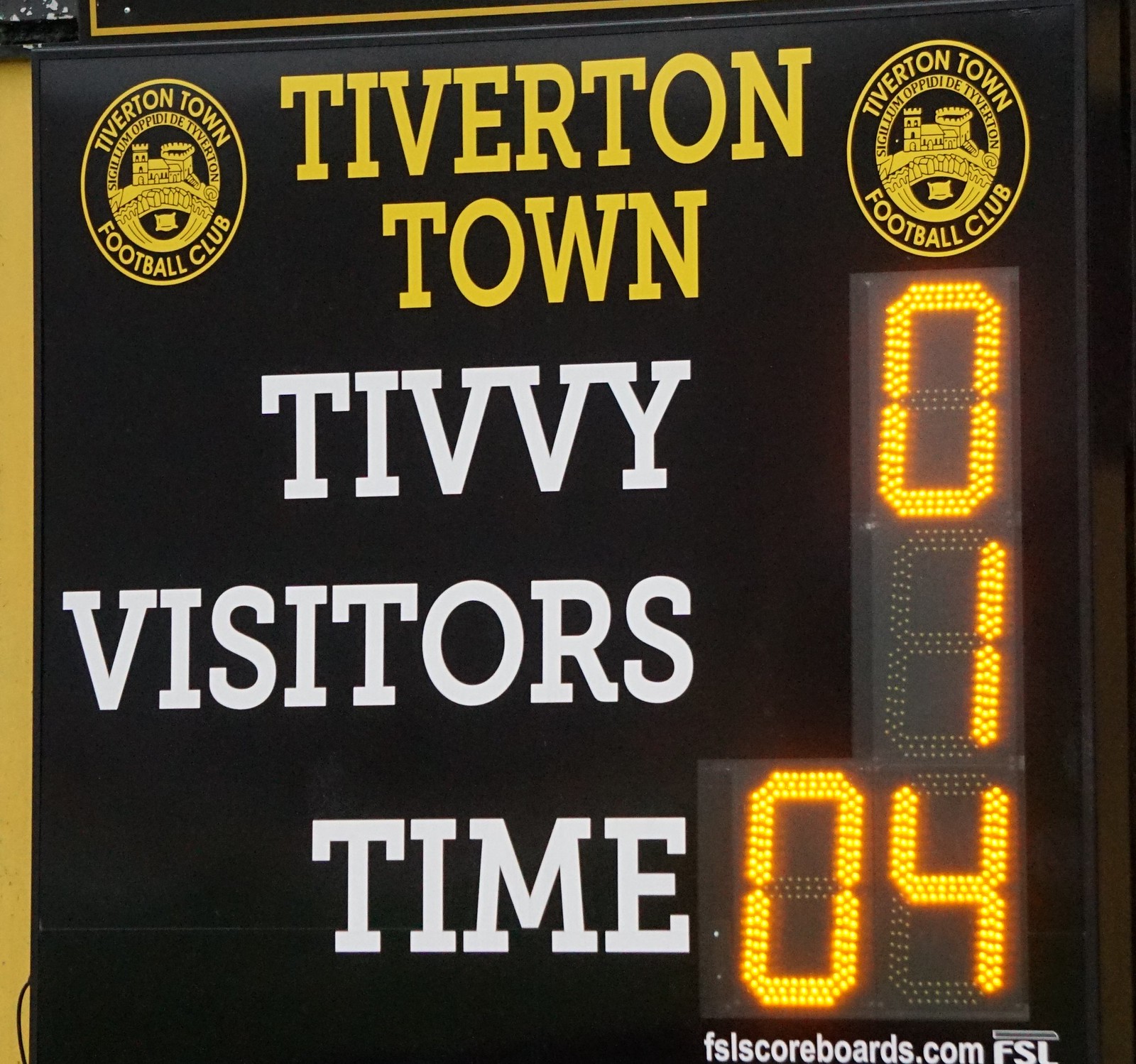The image depicts a predominantly black scoreboard with yellow and white text. At the top in bold yellow letters, it reads "Tiverton Town," flanked on either side by circular seals. Each seal says "Tiverton Town Football Club" and features an image of a castle with a bridge. Below the main title, in white letters, it reads "Tivvy" (T-I-V-V-Y), followed by the scores: “Tivvy 0” on the left side and “Visitors 1” on the right side. Further down, the word "Time" is displayed in white letters, with "04" indicating four seconds left on the clock. Additionally, "fslscoreboards.com, F-S-L" appears at the bottom right of the scoreboard. The entire setup is brightly illuminated, signaling its active use during a game.